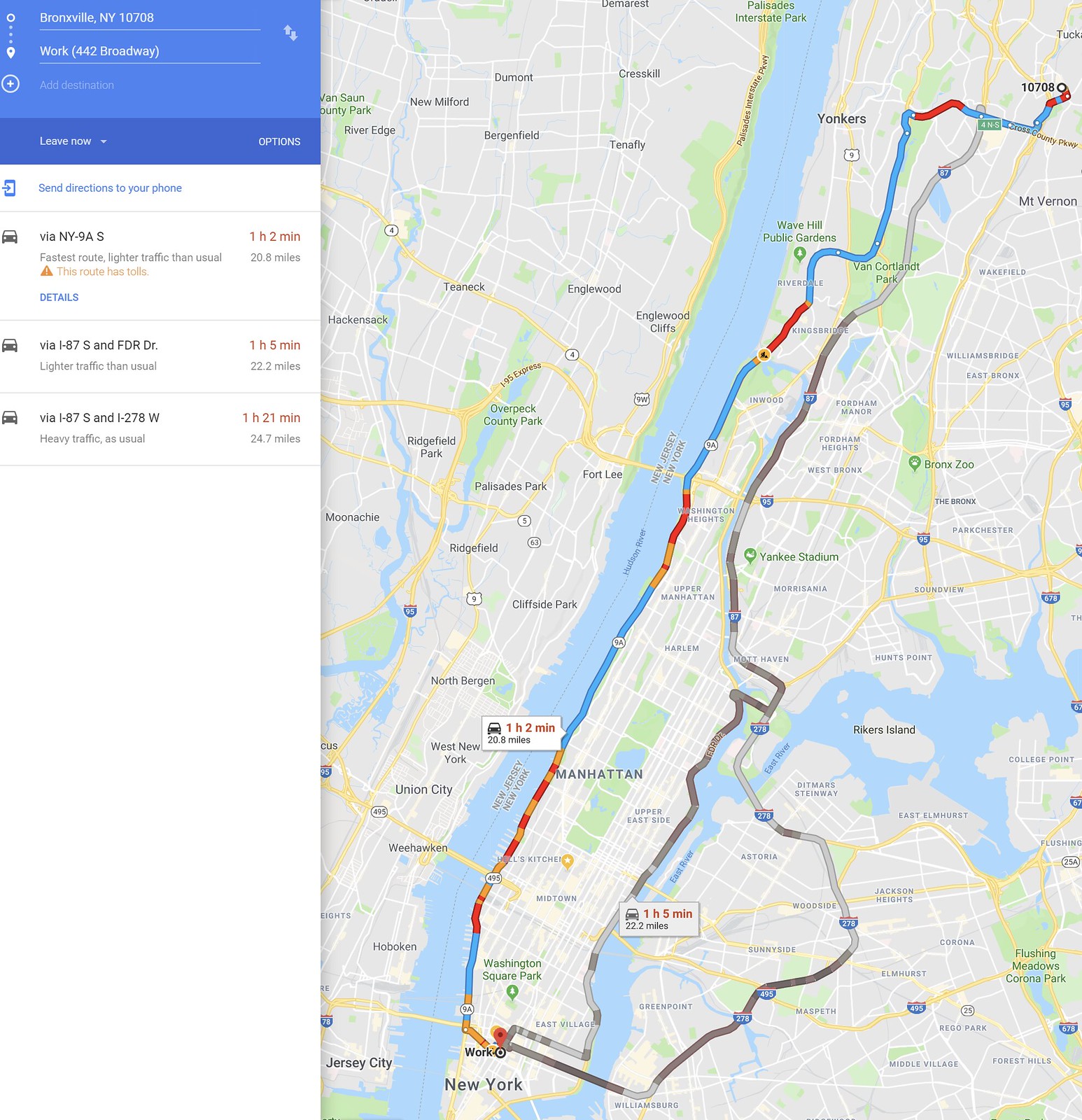A detailed caption for the image can be:

"A vivid color screenshot from a driving directions website showcases a map of New York City and its surrounding areas, focusing on a car trip that begins north of Mount Vernon and terminates in the heart of Manhattan. On the right-hand side, a vertical map prominently displays New York and Manhattan, with the Hudson River flowing vertically down the center at a slight angle. The map details three different routes to the destination. One route is highlighted in gray, while another is marked with segments in blue, yellow, and red, indicating different traffic conditions or route options. The left-hand side of the screenshot features a blue band, detailing that the journey starts from Bronxville, New York and ends at work located at 442 Broadway. It lists three route options: one via NY-NAS, another via I-87 South and FDR Drive, and the third via I-87 South and I-278 West. The overall clarity of the screenshot is impressive, with bright and distinct colors enhancing key details such as roads, routes, and landmarks. Notably, Rikers Island is also depicted on the map, adding to the geographic context."